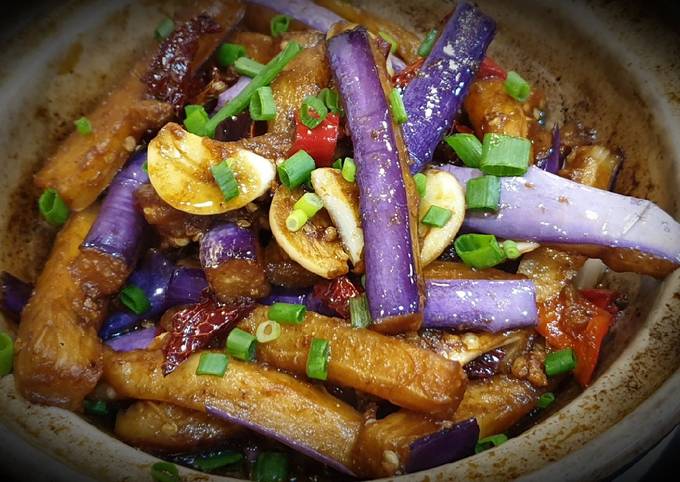This close-up photograph showcases a vibrant eggplant stir-fry elegantly plated in an earthen or clay pot. The dish features long, thin matchstick pieces of eggplant, about three to four inches in length, that are a striking bright purple with a glossy shine, indicating they've been sauteed. These eggplants are enveloped in a rich, shiny brown sauce or glaze, possibly soy sauce, giving them a slightly brownish hue. The dish is generously garnished with chopped green scallions and scattered with slices of garlic. Additionally, there are pieces of red chili peppers spread throughout, adding a hint of heat and color contrast. The visual and aromatic appeal of the dish, highlighted by these detailed ingredients, evokes the essence of East Asian cuisine, reminiscent of Chinese, Korean, or Japanese culinary traditions.